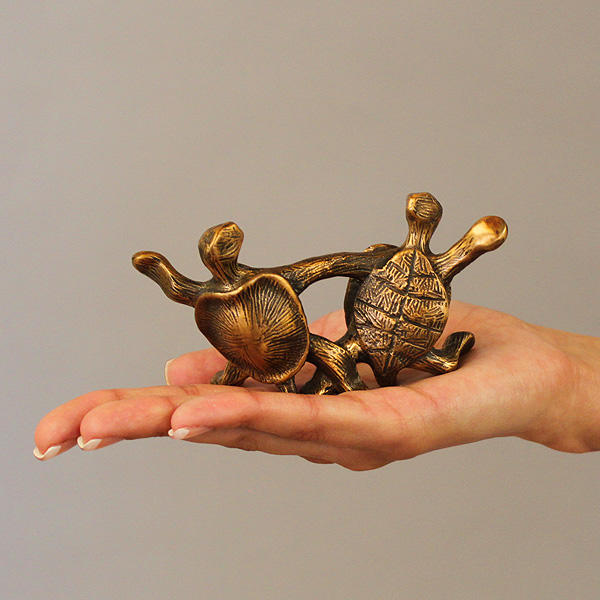The image captures an outstretched hand, palm facing upward, of a Caucasian woman with short, French-tipped manicured acrylic nails. The hand is holding a small, intricate bronze statue depicting two anatomically correct turtles in a dancing pose. The turtles stand on their hind legs, one with an arm outstretched behind while the other mirrors its partner, both holding one arm together as if in mid-dance. The bronze sculpture features a brushed texture, creating a shiny and brown patina throughout. The turtles' shells differ slightly, with one showcasing a block pattern and the other having smoother lines. The artwork combines elements of whimsy and realism, emphasizing the turtles' elongated limbs and detailed texturing.